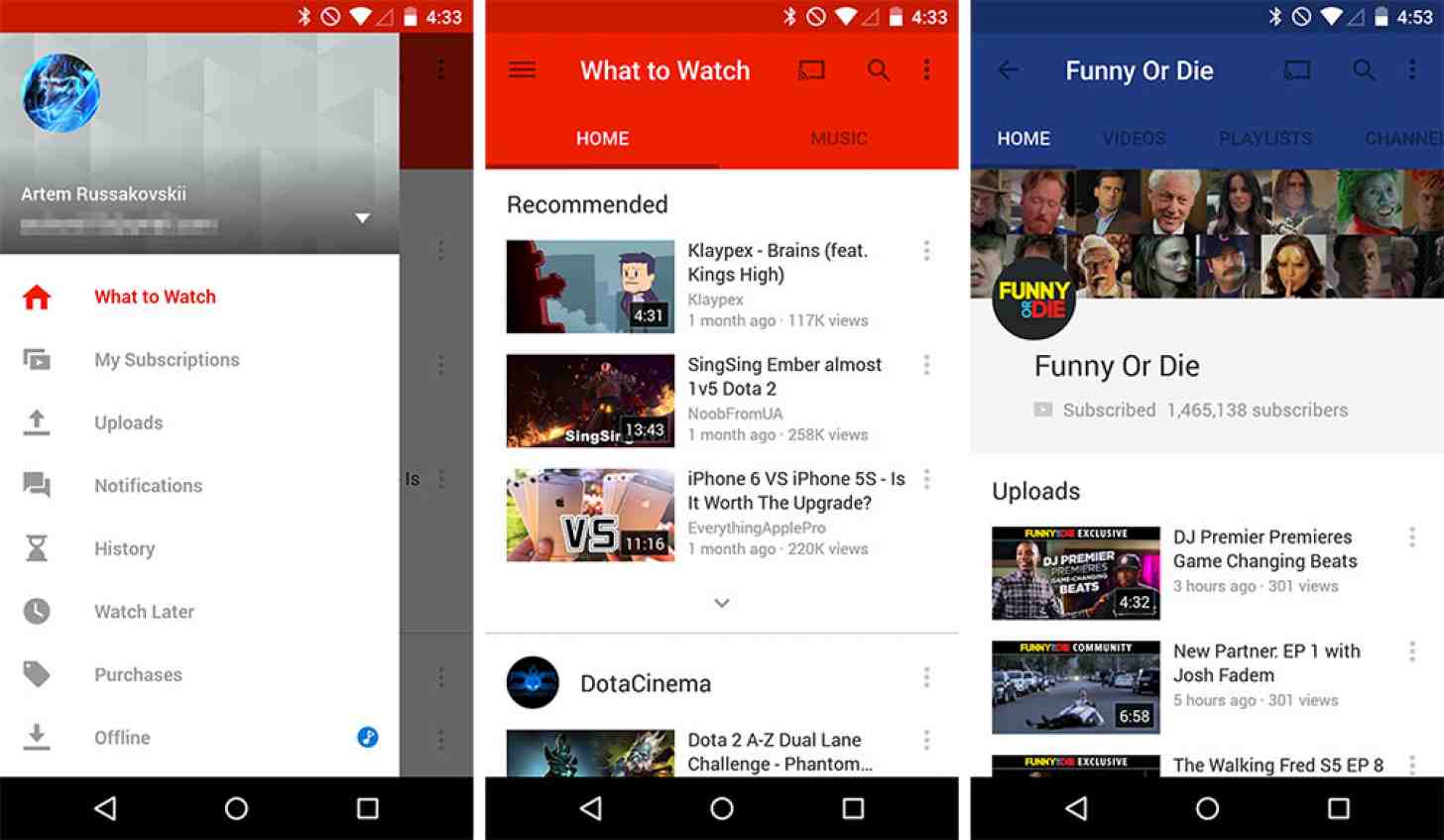The image features three smartphone screenshots displayed side by side. 

**First Screenshot:** 
The device displays the time as 4:33 PM with a half-full battery and a strong Wi-Fi signal. The screen showcases a profile under the name "Artem Russakovsky" with a prominent blue-themed picture. Beneath the name, there are various options including "What to Watch," "My Subscriptions," "Uploads," "Notifications," "History," "Watch Later," "Purchases," and "Offline." Playback controls featuring play, rewind, and stop icons are visible. The user has selected the "What to Watch" tab.

**Second Screenshot:** 
This screen shows the "What to Watch" page, populated with three video recommendations:
1. "Klaipax Brains," streamed one month ago with 117,000 views.
2. "Sing Sing Ember, Almost."
3. "iPhone 6 vs. iPhone 5s: Is it Worth the Upgrade?"

**Third Screenshot:** 
The final image is dedicated to the "Funny or Die" channel, to which the user is subscribed. The channel boasts 1,465,138 subscribers and showcases three recent uploads.

Through these detailed screenshots, the viewer gains insight into the user's video browsing and subscription preferences.